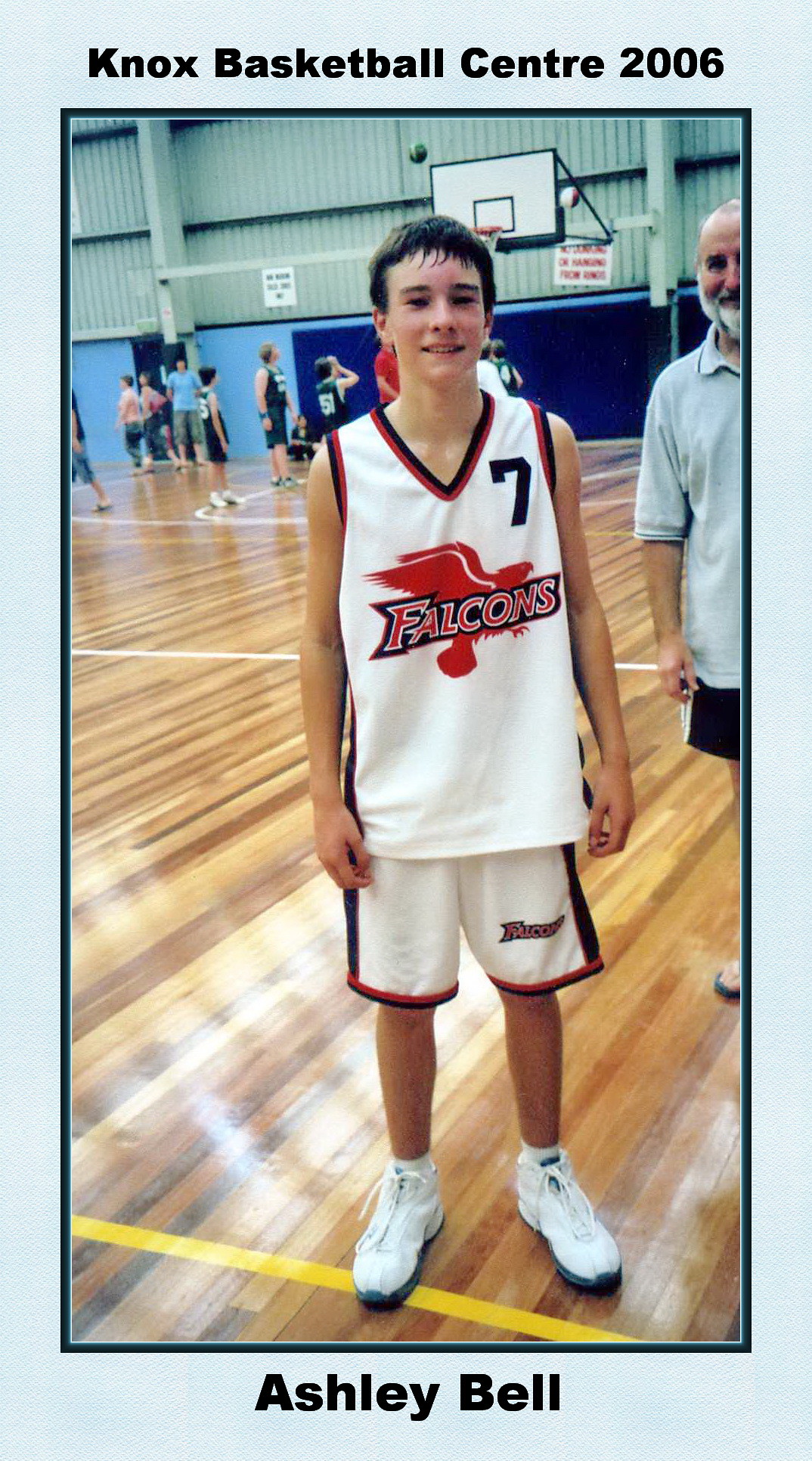This detailed photograph resembles a sports card, prominently showcasing a young basketball player, likely in junior high or high school, in the midst of a game on an indoor court. The image, framed by a light blue border, has text above and below. At the top of the border, in black text, it reads "Knox Basketball Center 2006," and the bottom text reads "Ashley Bell," likely indicating the player's name.

The central subject, Ashley Bell, is a young male with black hair, visibly sweaty from play. He dons a white basketball jersey with red and black accents, emblazoned with the word "Falcons" in a stylized font featuring a red falcon outline. The jersey also bears the number seven. His matching shorts and white shoes complete his athletic attire. Bell stands at the center, smiling as though posing for the camera, amidst active gameplay. In the background, several players can be seen, including a basketball seemingly heading toward a hoop. To the right, partially cropped out, is an older man dressed in a blue shirt with a beard, further adding context to the scene.